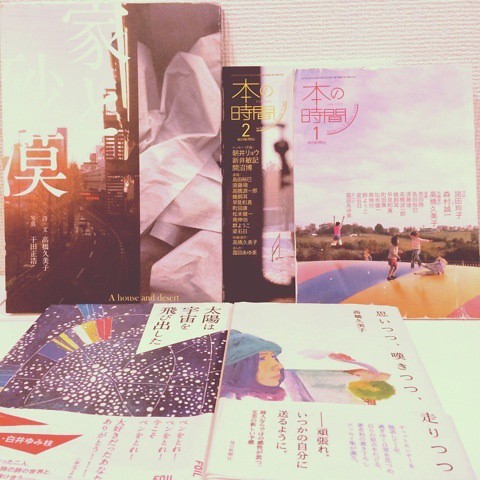The image depicts a tightly-cropped, organized display of various Japanese books and pamphlets, all adorned with traditional vertical Japanese script. Situated atop what appears to be a white textured cloth covering a table, five to six items are conspicuously arranged. In the background, several books stand upright, partially overlapping each other, creating a bustling showcase-like atmosphere. Two prominent books lie flat in the foreground.

One of the standing books features a cityscape under bright sunlight, characterized by buildings and traditional Japanese characters. Another showcases children energetically playing and jumping on a multicolored, striped surface, seemingly an inflatable structure, with a vibrant outdoor setting of blue sky and grassy fields. A third contains an illustration of a woman wearing a blue hat, gazing into the distance, embellished with red Japanese text. There is also mention of a book with a visually appealing starry sky, imbued with vibrant hues of oranges, yellows, and blues.

The foreground books include one predominantly adorned in black and white with gold markings, partially covered by the image of children. Another displays intricate designs with a collage of papers and images, including circles of green, yellow, and blue. The precise setting—whether a bookstore or a personal collection—is left ambiguous, as the closely cropped image leaves the surrounding environment to the imagination. The vibrant and diverse imagery on the books, from cityscapes to playful children and contemplative figures, collectively portray a rich tapestry of Japanese cultural elements.